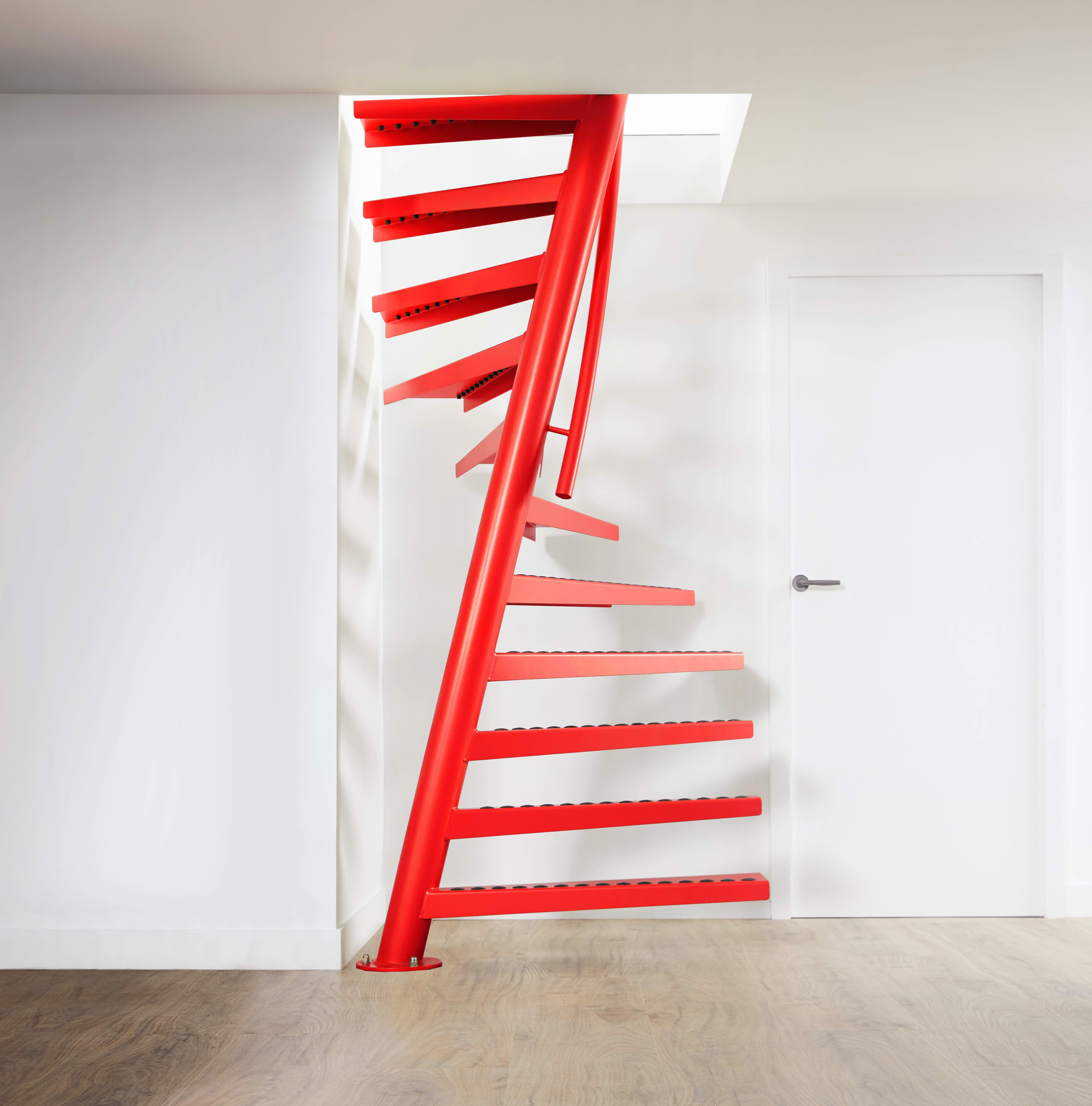The image depicts a modern, minimalist room with pristine white walls and a very white ceiling. On the right-hand side, there is a closed white door equipped with a gray handle. The floor is adorned with contemporary fake wooden laminate in a brownish hue. The central focal point of the room is an eye-catching, bright red spiral staircase that ascends towards a skylight. The staircase, supported by a red pole running diagonally from left to right, features steps resembling flat, textured Legos with large circular holes throughout. The lower portion of the staircase lacks a railing, though a railing appears about halfway up. The staircase’s artistic and modern design gives it a sculptural appearance, seeming as though it's suspended in the space.